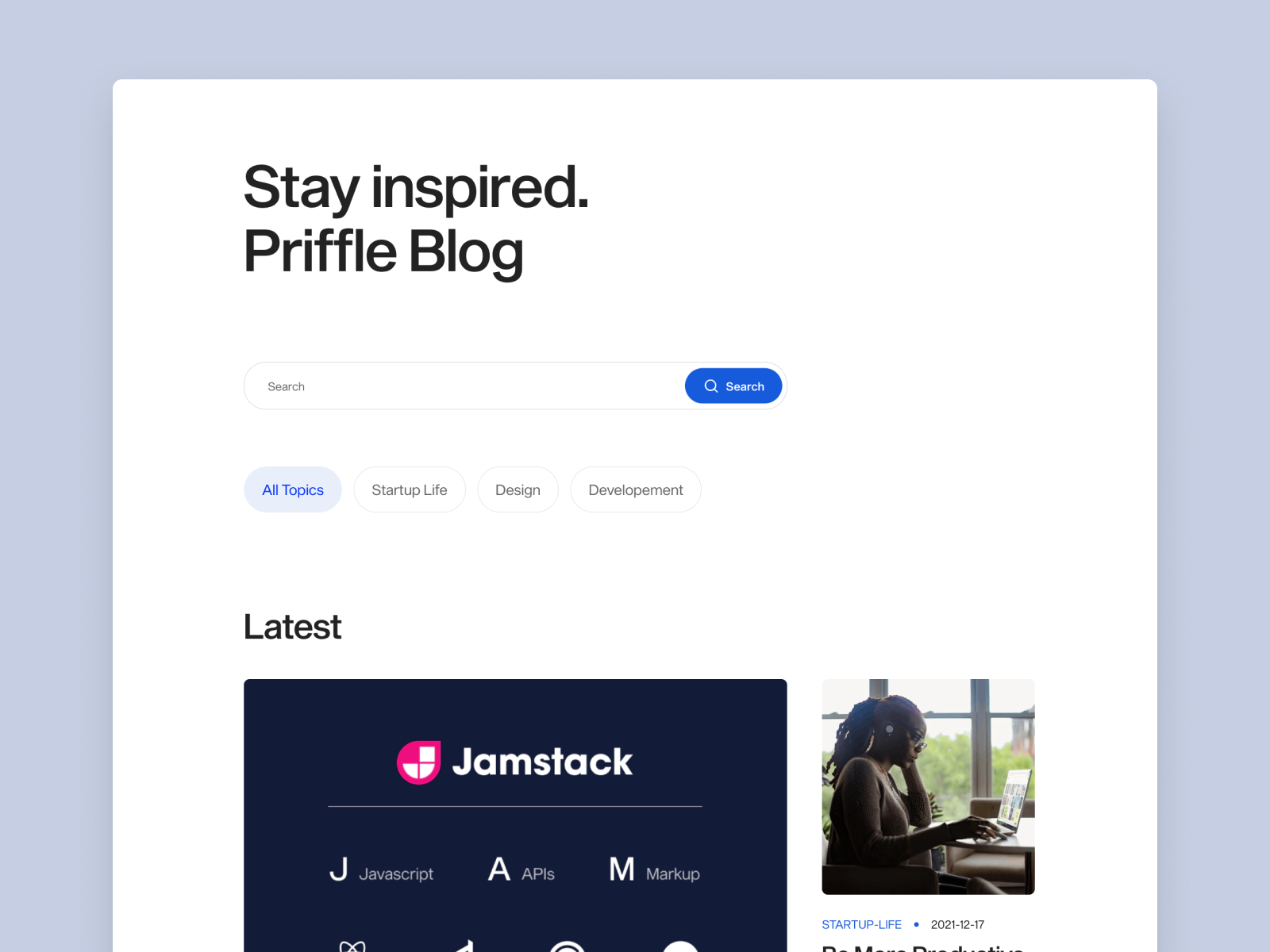A detailed screenshot of a website landing page is set against a gray background. The main website body, displayed within a large white area, features a header in the top left that reads "Stay Inspired Cripple Blog" in bold black text. Directly below the header is a search bar with a blue oval button labeled "Search" in white, accompanied by a magnifying glass icon on the right side of the bar. Beneath the search bar, four navigation tabs are listed as "All Topics," "Startup Life," "Design," and "Development."

On the left side of the landing page, the heading "Latest" appears in large, bold black letters. Under this heading, a black rectangle displays a pink and white logo with the letter "J." To the right of the logo, the word "JAMstack" is presented in white text with an underline. The acronym JAM is explained in smaller text to the left, signifying "JavaScript," "APIs," and "Markup," each word starting with an uppercase letter corresponding to JAM.

Partially cut off at the bottom edge, several icons are just visible but indiscernible. On the right side of the image, a woman in her 30s is seated at a round table in an office environment. She is working on a laptop and facing to the right. The office features large windows in the background. Below this segment, the text "Startup Life 2021-12-17" provides a timestamp or date reference.